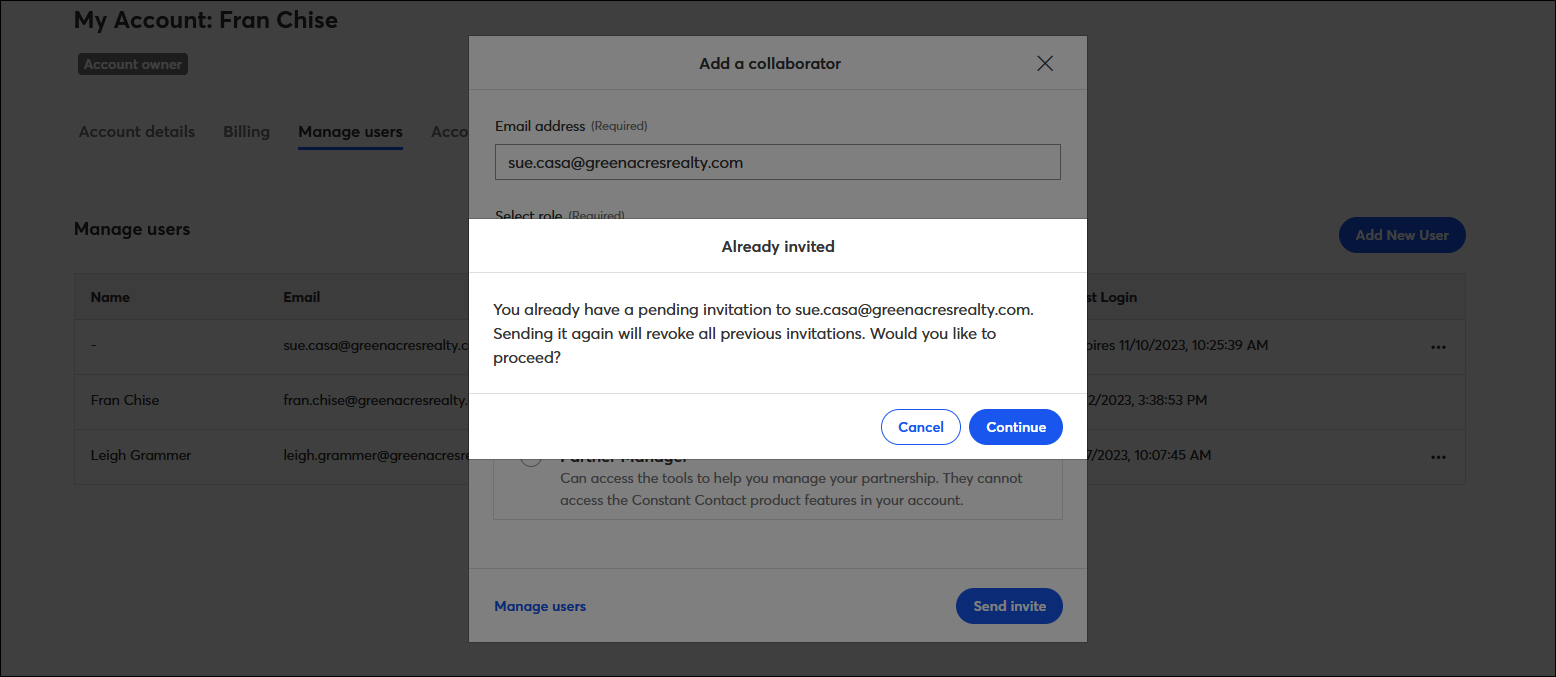The image depicts a website interface with a dark gray overlay. In the background, the 'My Account' section is visible, belonging to a user named Francis. Various elements on the screen are highlighted in boxes. A notable section displays the option to 'Add a Collaborator' via an email address. The overlay warns that a pending invitation already exists and sending a new one will revoke previous invitations, giving the choices to either 'Cancel' or 'Continue'. The action options are prominently displayed in a white box with dark lettering, contrasting against the lighter gray insert. At the bottom, there's a disabled comment section, indicating the user is unable to proceed with additional remarks due to their current focus on synchronizing team activities. The overall aim appears to be resolving an issue to return to the regular site interface.